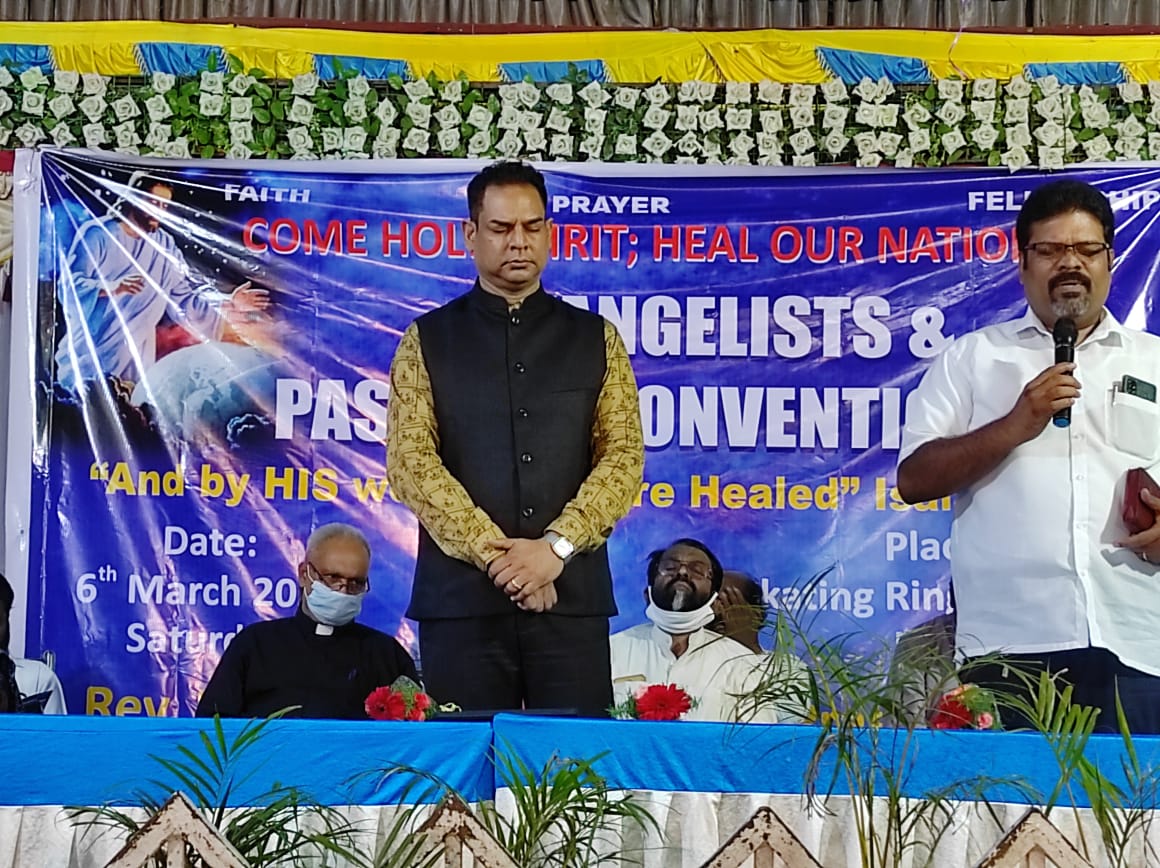In this detailed rectangular image, a man is seen performing a religious ceremony. He stands in front of a large blue laminated sign with a blue gradient background. The top left corner of the sign features an illustration of a Jesus-like figure surrounded by stars. Above the sign, tiny rose-like objects in light green line the space beneath a bright yellow and blue curtain. The central figure is a man dressed in a black vest and black pants, wearing a long-sleeved shirt that is light brown with dark brown detailing, along with a silver watch and a wedding ring. His eyes are closed, and he holds his hands together in a prayerful gesture.

To his right stands another man in a white button-up shirt and glasses, holding a microphone and a smartphone in his front shirt pocket. He appears to be praying with his eyes closed. Behind these two men, there are four seated individuals also engaged in prayer. The backdrop is a banner that reads, "Come Holy Spirit, Heal Our Nation, Evangelists Pastor Convention," with the date "6th March" displayed. The scene gives an impression of a solemn religious gathering, possibly involving people of Indian heritage, focused on prayer and spiritual reflection.